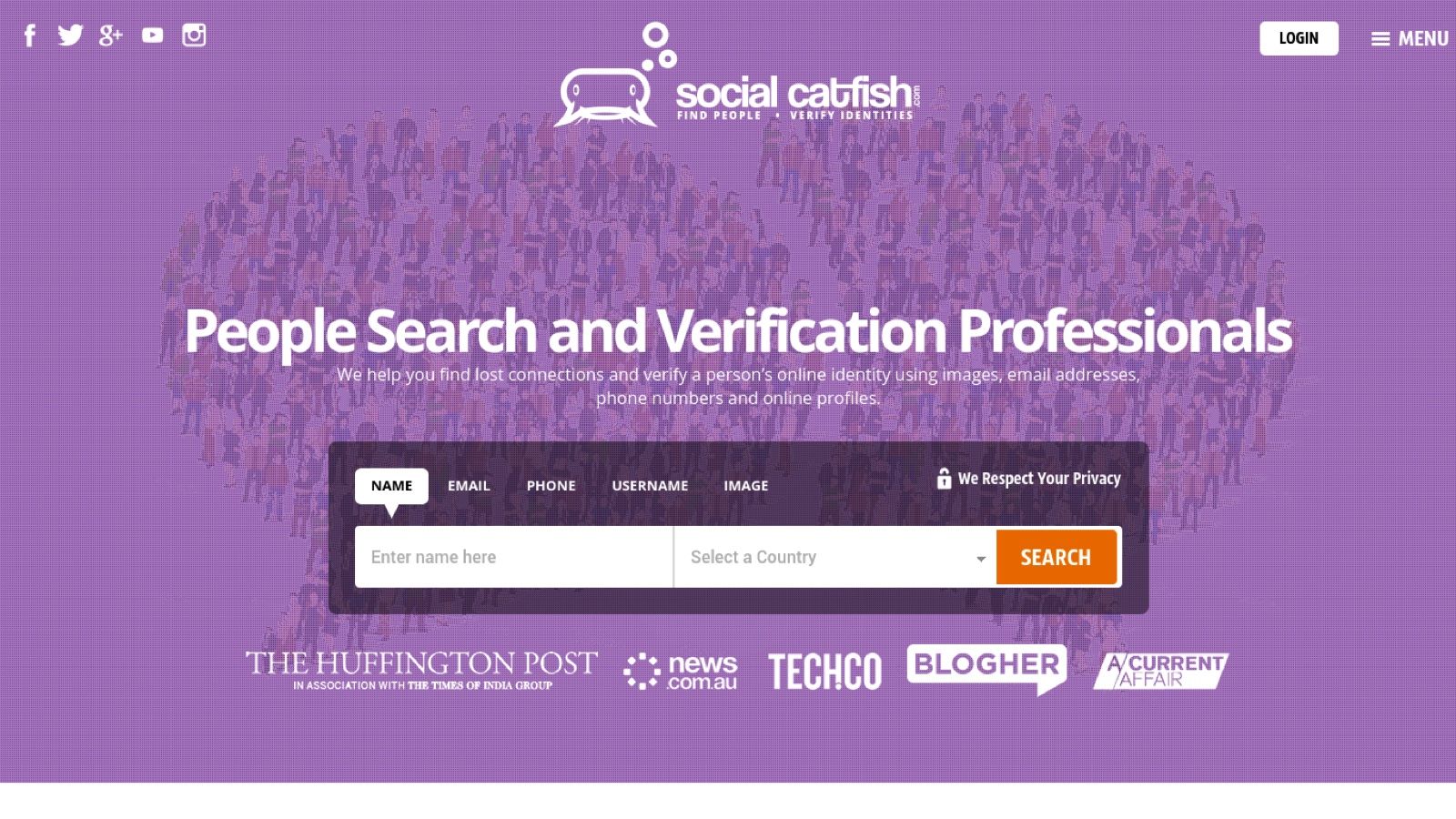The image is a detailed screenshot from a website. In the upper right-hand corner, there is a menu button represented by three horizontal lines indicating a dropdown menu. Adjacent to it is a rectangular, white "Login" button with black text. 

The center of the screen features a distinctive catfish logo with three bubbles emanating from its head. Beside the logo, the text reads: "Social Catfish: Find People, Verify Identities."

The upper left-hand corner displays icons for various social media platforms: Facebook, Twitter, Google+, YouTube, and Instagram.

The background of the image is a purple hue, featuring a logo composed of several people standing and conversing with one another. Overlaying this, there appear to be two word bubbles colliding, though the visual is partially obscured by text and interface elements.

Dominating the center of the screen, in large white text, it reads: "People Search and Verification Professionals." Below this headline is a darker rectangular search box with the label "Name" highlighted. Users are prompted to "Enter Name Here" and select a country before clicking an orange "Search" button.